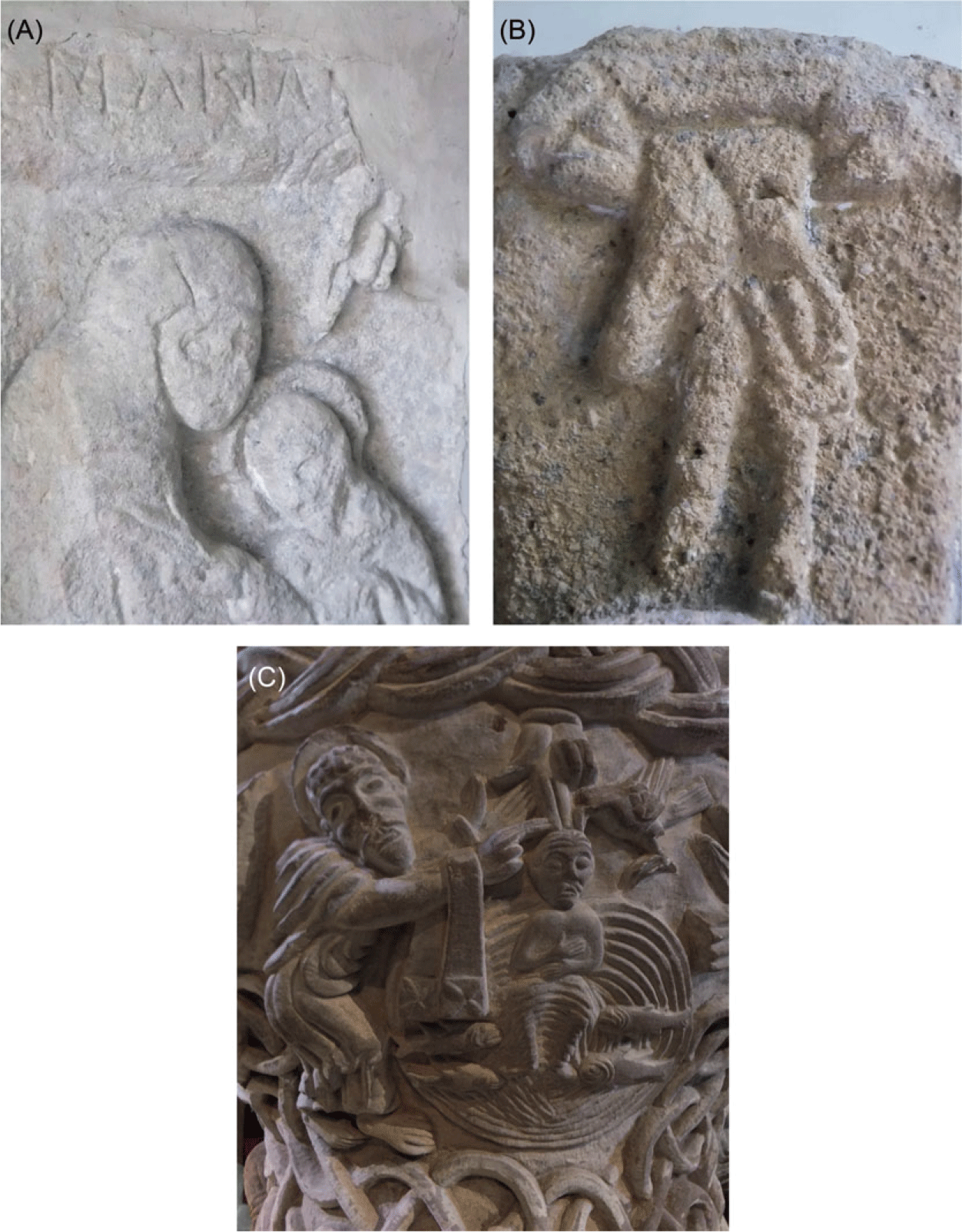The image features three photographs of ancient bas-relief sculptures labeled A, B, and C, each carved into stone. Picture A, located at the top left, depicts a simplistic figure which appears to represent two people, likely a mother and child, with faintly carved letters "M, A, M, A" above them. The figures are basic and relatively unsophisticated, showing just their heads and shoulders. Picture B, situated at the top right, is significantly more eroded and harder to interpret. It resembles a hand making a gesture, possibly a peace sign, carved into deteriorating stone, making the exact form difficult to identify. Picture C, positioned below A and B, portrays a slightly more detailed scene of a bearded man attending to a small child, possibly fixing the child’s hair. This carving is richer in surface texture and decoration compared to the other two, suggesting it could be part of a medieval stone pillar or cathedral detail. All sculptures exhibit a weathered and gray stone color, indicating their ancient origins.